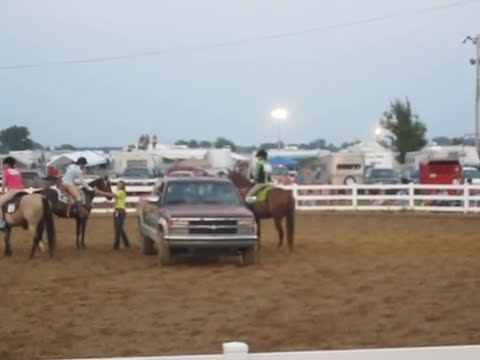The image depicts a dirt corral at a horse ranch, enclosed by a waist-high white fence. In the center of the corral, there is a maroon-colored Ford pickup truck with its front facing the camera. Surrounding the truck, three horses, two brown and one light beige with a dark tail, stand with their riders. On the right side of the truck, a rich brown horse is stationed, while on the left, a dark brown horse is positioned nearer to the truck, and a light beige horse is further left. A person on the ground in front of the horses appears to be communicating with the riders. In the background, beyond the fence, various buildings, RVs, and horse trailers are visible. Distant treetops form a horizon line under a hazy gray sky, with an electrical pole and line stretching across. A single tower with a bright light on top stands illuminated far off in the distance. Overall, the setting has a slightly dusty, late afternoon or early evening ambiance.